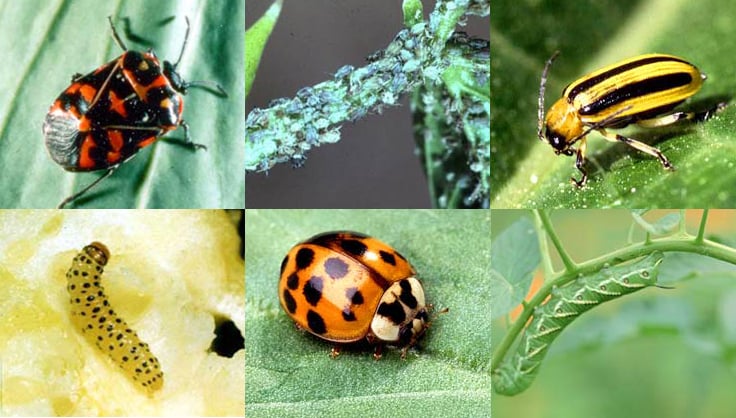The composite image features six highly detailed and colorful photographs of different insects, arranged in three columns and two rows. The top left shows a close-up of a black and orange beetle-like bug resting on a leaf, its intricate details clearly visible. In the top middle image, a long stem is covered with numerous small black and gray ant-like bugs. The top right image depicts a yellow and black striped bee-like bug perched on a green leaf, showcasing its antennae and two visible legs. On the bottom left, there is a tiny yellow caterpillar with black spots on a yellowish surface, emphasizing its segmented body. The bottom middle photo captures a ladybug-esque insect with an orange shell and dark splotches, positioned on a green leaf. The bottom right image displays a green caterpillar with white diagonal stripes, climbing up a curved green stem. The images are vivid, magnified, and arranged without any accompanying text, making them suitable for educational purposes such as in textbooks or insect guides.